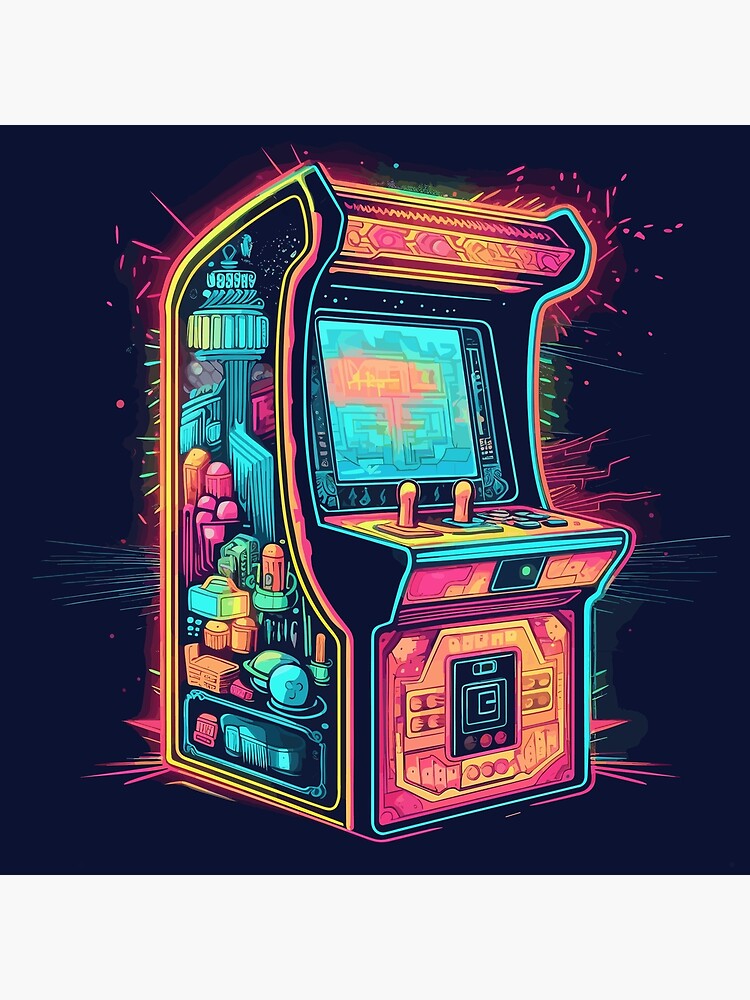The image portrays a vividly detailed digital artwork of an arcade cabinet against a navy blue night sky background. The arcade game, prominently placed slightly left of center, features a retro-futuristic design with its left side intricately decorated with tech gadget graphics and circuit board patterns in a spectrum of colors including orange, pink, purple, and teal blue. The front of the cabinet showcases a large blue teal square screen with a hint of orange at the center, flanked by two orange joysticks and a set of teal buttons to the right. Below, the coin slot area is defined by a black square with a teal outline, surrounded by an orange and red gradient. The arcade cabinet has a unique boxy shape, flaring out at the top, and is accented with various shapes and designs in bright hues of yellow, pink, and green. Red sparks emanate from the cabinet's corners adding to its dynamic appearance. Overall, the artwork captures the essence of a unique, retro, and vibrant arcade experience, with the dark blue backdrop enhancing the energy radiating from the machine.